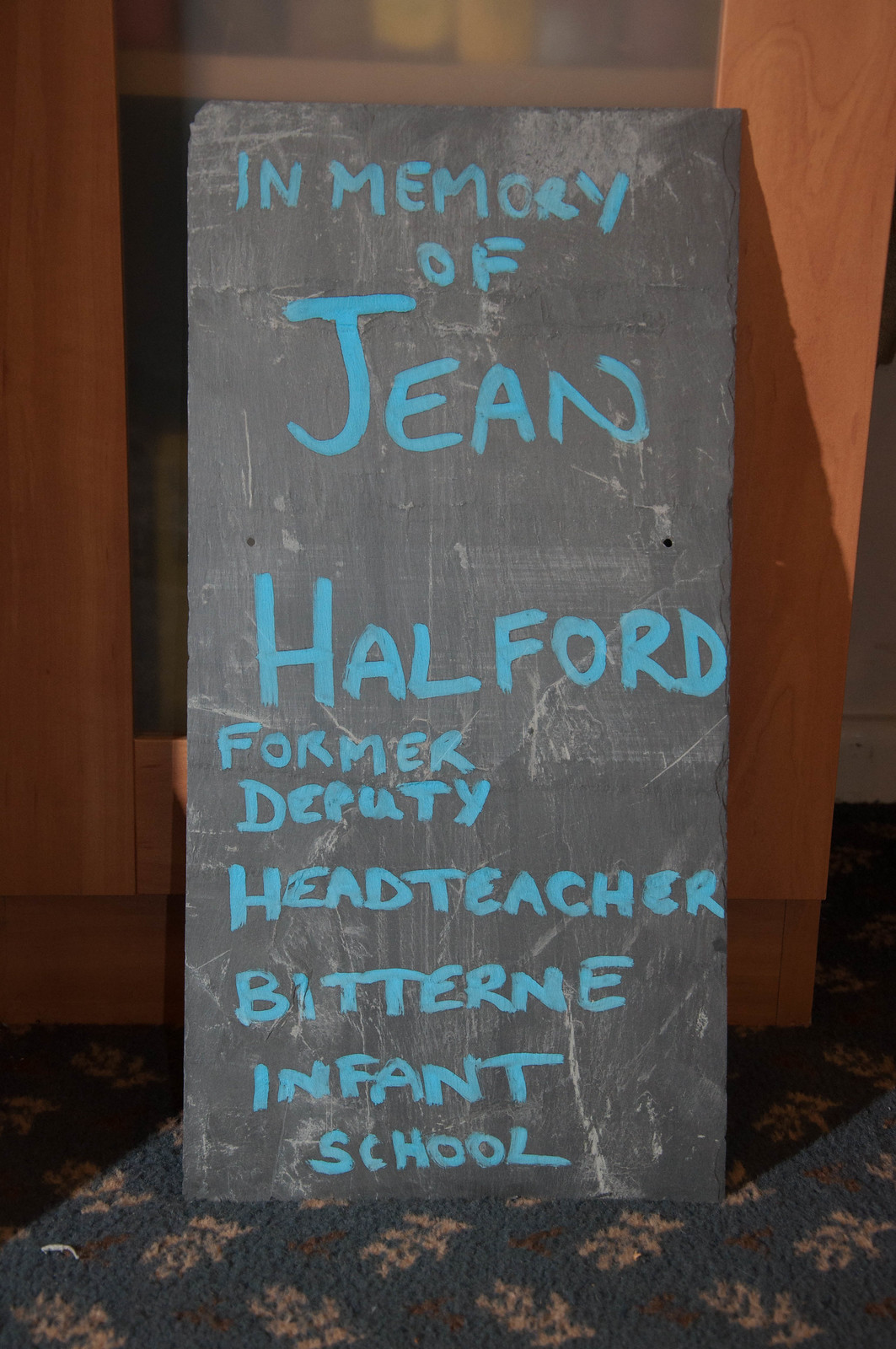The photograph features a large, dark gray, rectangular slate board with white smudge marks, giving it a natural, earthy texture. This board, positioned squarely in the center of the image, leans against a light brown wooden cupboard, which has an opaque glass panel in its middle, revealing a shelf with various items. The slate has inscriptions in blue, hand-written text in memory of Jean Halford, with "Jean Halford" prominently bolded. The full text reads, "In memory of Jean Halford, former deputy head teacher, Bitterne Infant School." The board rests on a multi-colored carpet with a blue and white pattern, enhancing the cozy, indoor setting which appears to be inside a house, suggesting a quiet tribute to Jean Halford's legacy.